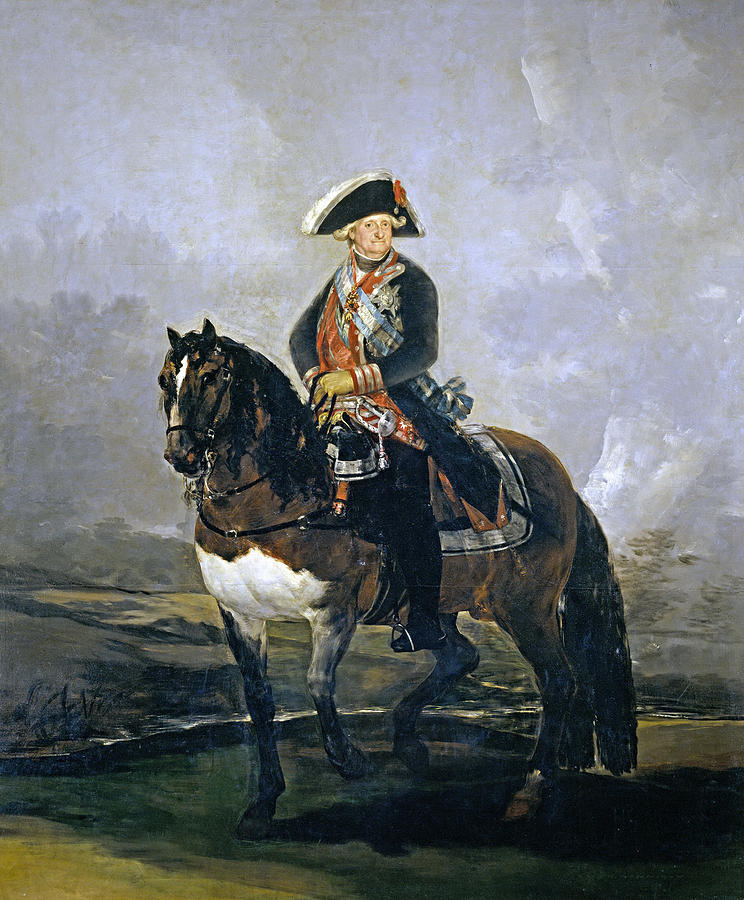This is an oil painting created by Francisco de Goya around 1800, titled "Charles IV on Horseback." The portrait-oriented artwork vividly portrays a military officer seated on a brown horse, which sports a distinct white chest. The officer, who resembles historical figures like Napoleon or George Washington, is dressed in a detailed military uniform. The outfit includes a dark blue jacket with gold-striped cuffs, a red vest, black pants, and a triangular dark blue hat adorned with white trim and a red flourish. Underneath the hat, a silver-white curly wig is visible. The officer's uniform features a silver sash across his shoulder, and he is decorated with numerous badges and ribbons. The horse and rider dominate about two-thirds of the image from left to right. Behind them, the background showcases a rugged, green hilly terrain, under a stormy, bluish-gray sky filled with fluffy clouds. The painting exemplifies the Romanticism style with its dramatic use of color and attention to detail.